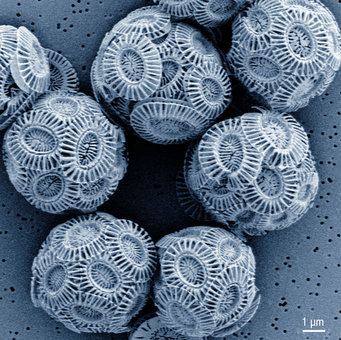This detailed image, likely taken through a microscope, shows a collection of intricately patterned, bluish-gray circular objects resembling balls, possibly composed of fine spiny structures layered to form spherical shapes. Six of these balls are fully visible, while two appear partially cut off at the top and left edges of the frame. The objects rest on a porous, gray surface dotted with small holes, reminiscent of a cheese-like texture. The balls exhibit numerous lines and circular patterns, giving them a firm yet potentially fuzzy appearance. A watermark or signature featuring the symbol "1 µm" (micron) is visible in the bottom right corner, indicating the scale of the image.